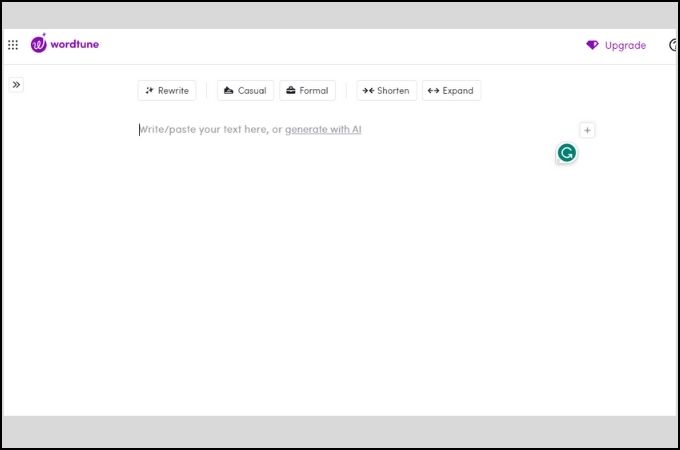The image depicts a desktop application or app interface named WordTune. The interface features a predominantly purple color scheme, with a distinct "W" logo positioned in the upper left corner. In the upper right corner, there is an "Upgrade" option highlighted in purple with a diamond icon beside it, accompanied by a small question mark for additional information. 

The main workspace of the interface is largely white, with various sections dedicated to different text modification options, such as "Rewrite," "Casual," "Formal," "Shorten," or "Expand." A placeholder text within this area prompts the user to "Write or paste your text here or generate with AI," and there is a small "G" icon whose function is unclear. 

The bottom portion of the interface is shaded in a darker gray. Additionally, there is a plus icon next to the "write or paste your text" area and a double forward arrow tab indicating further functionalities. The image suggests that WordTune is designed to assist users with text editing, potentially offering services to refine grammar or improve writing style. The workspace is currently blank with no text pasted or written in the provided fields.